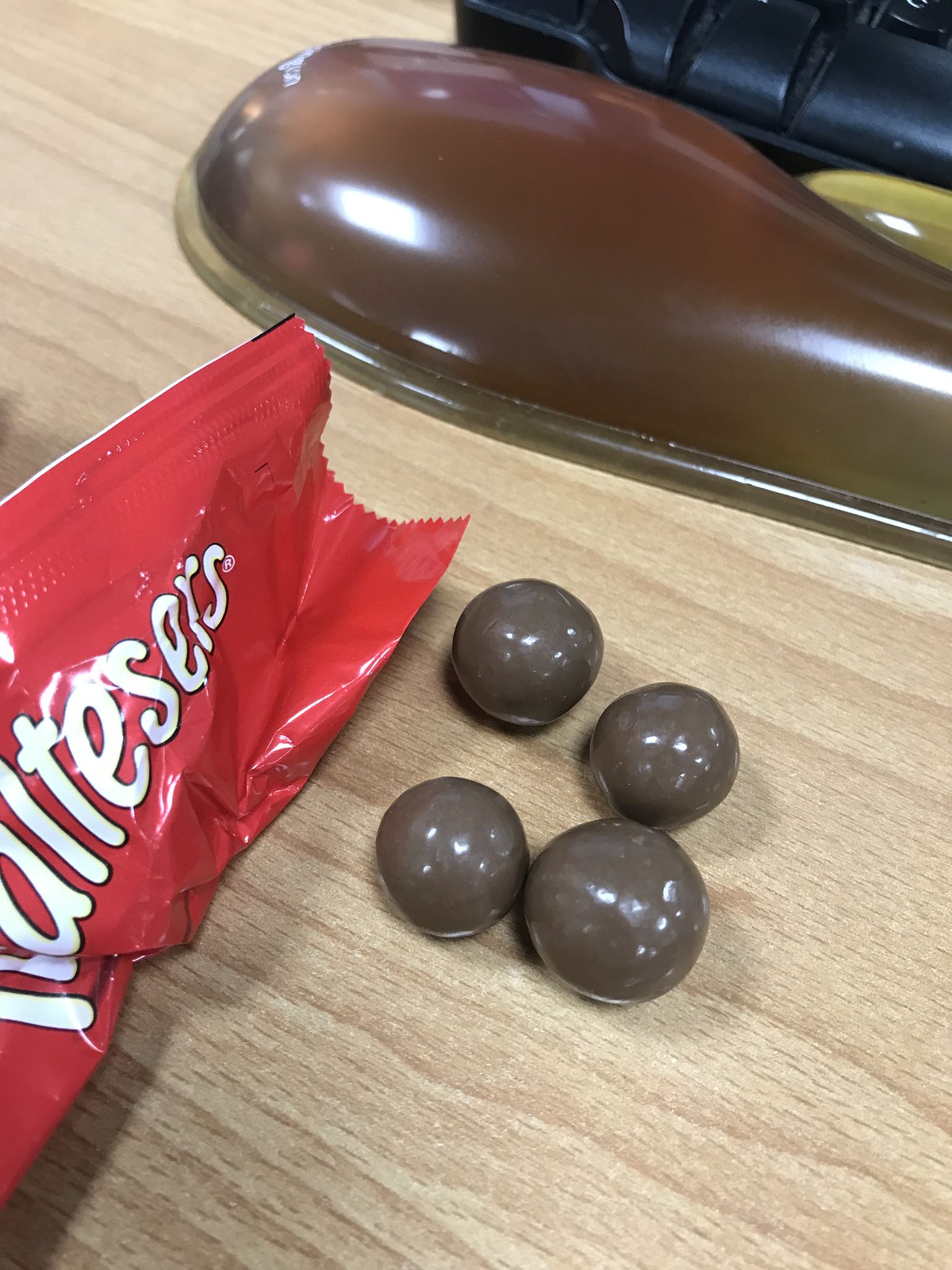The color photograph in portrait mode showcases four malted milk balls, each coated in a shiny brown chocolate layer, resting directly on a light wooden surface. Prominent in the image is a wrinkled red wrapper featuring partially visible white and cream-yellow writing, positioned to the left of the candy, though the text remains unreadable due to cropping. Arranged with one slightly larger piece at the bottom, the balls are symmetrically positioned with one to its left, another touching the top edge, and the last slightly further left again. In the blurry background, there is an indistinguishable plastic, oblong circular object with white writing, alongside another black, plastic, rounded object, both partially visible. The dynamic composition places emphasis on the malt balls, their glossy chocolate coating glistening against the rustic wooden backdrop.